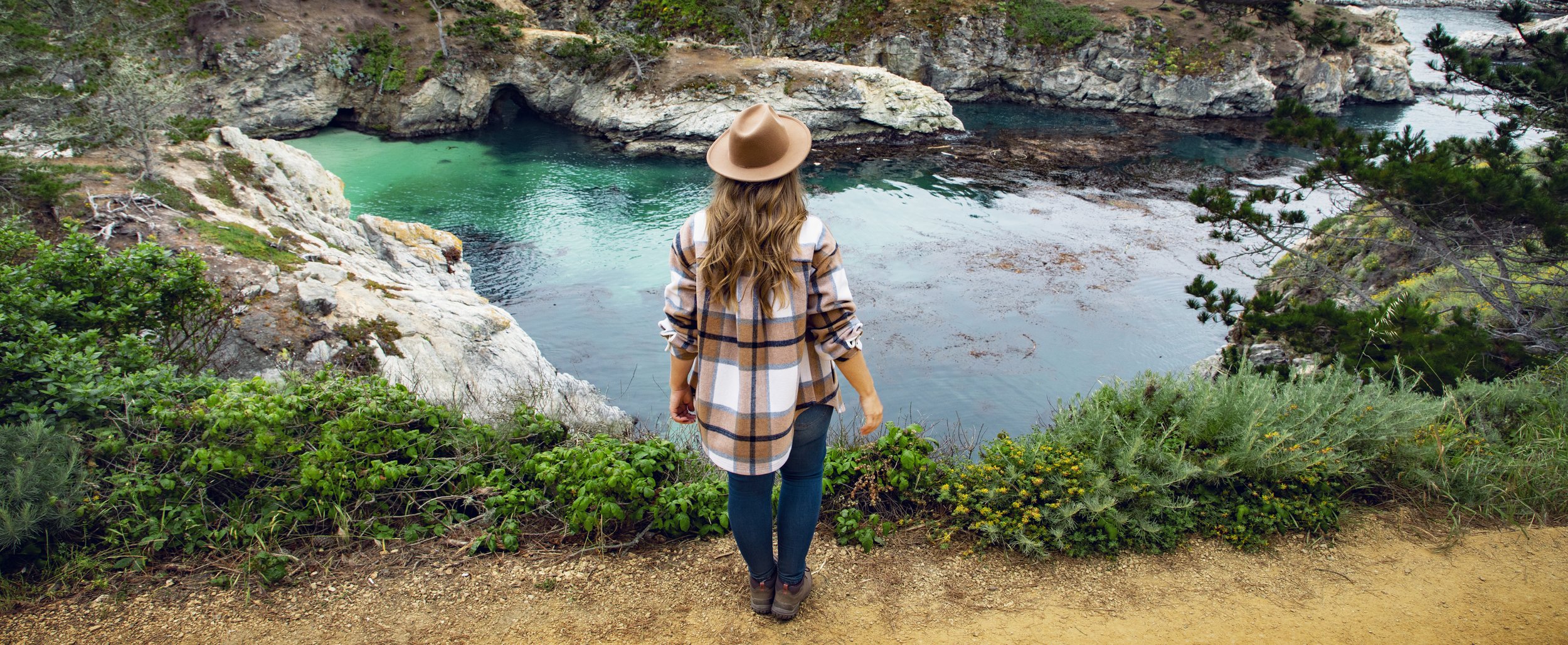This wide rectangular photograph captures a serene nature scene with a woman standing on a trail overlooking a river. The woman, centrally positioned with her back to the camera, wears a brown wide-brimmed hat and a detailed flannel shirt featuring a pattern of browns, whites, light browns, and black lines. Her tight blue jeans and brown boots complete her outfit. Her wavy, blondish-auburn hair cascades down her back. 

She's facing a river several meters below the elevated path she stands on. The river's clear, greenish-blue waters flow gently, displaying patches of brownish algae and submerged rocks. Surrounding the riverbanks and cliff faces are striking whitish-grey rocks, some tinged with yellow, and a variety of green mossy shrubs. On the river's left bank, noticeable cliff faces have a small cave nestled among them. Verdant greenery and trees spread out across the scene, with some branches poking in on the right side of the image. This combination of elements enhances the picturesque landscape, casting a tranquil and immersive atmosphere.